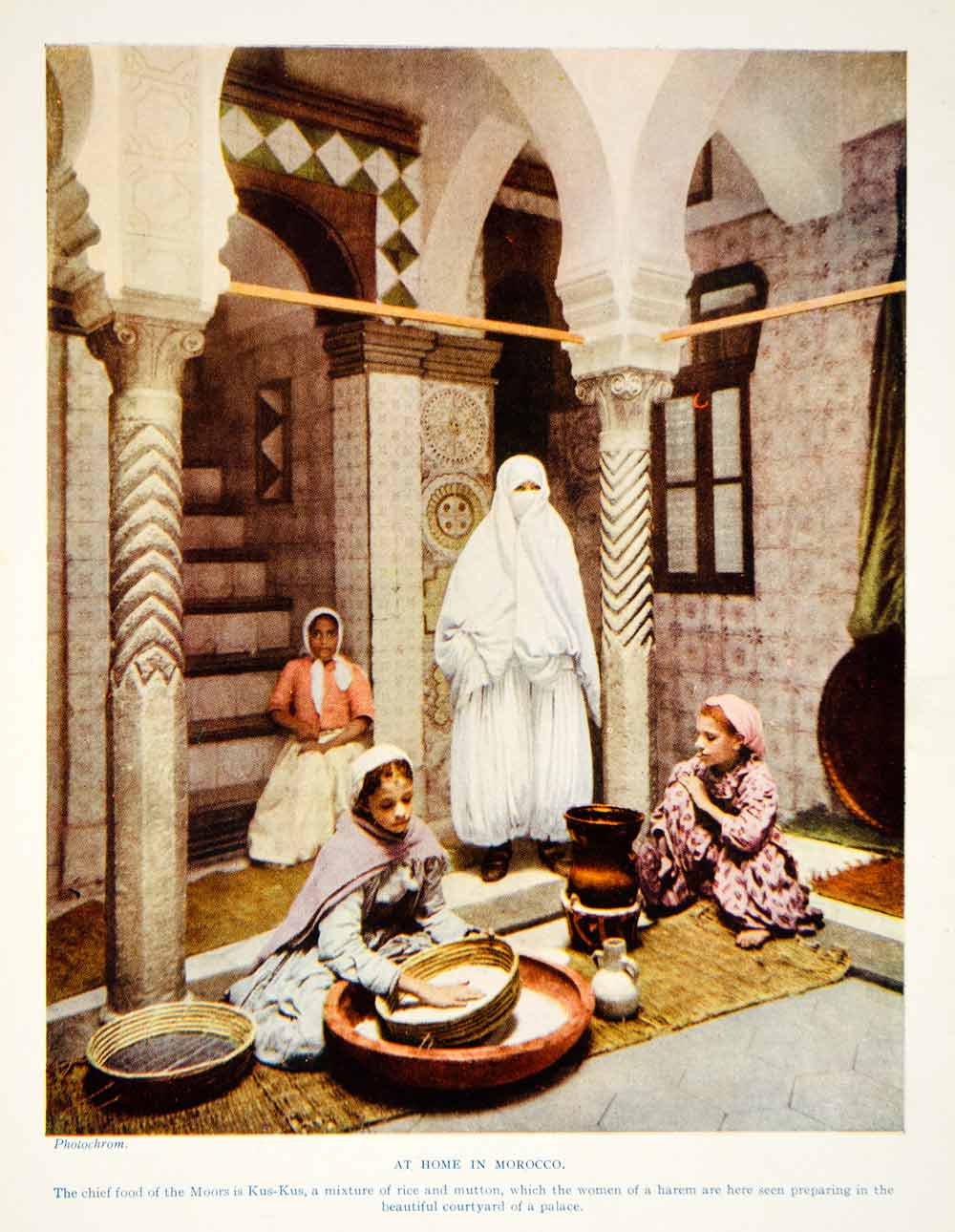The image appears to be a poster or a page from a magazine, possibly National Geographic, depicting a beautifully detailed courtyard in a Moroccan palace. This courtyard is adorned with intricately designed tiles and mosaics, accompanied by elegant columns and arches in multiple colors. The room is spacious and visually stunning, with a blend of traditional Middle Eastern architectural elements. 

In the scene, four women are preparing couscous, a traditional Moorish dish made of rice and mutton. Three women are sitting or kneeling on woven straw mats, engaged in the preparation. One woman, dressed in a vibrant pink outfit, is squatting, while another, wearing an orange blouse and white skirt, is standing and possibly assisting. The third woman, clad in a headscarf that leaves her face visible, is working with large bowls and wicker baskets. All three have some form of loose hijab revealing parts of their hair.

In the background, a fourth woman dressed entirely in white stands, with only her eyes visible through a burqa, adding a solemn presence to the bustling activity. This figure underscores the cultural and traditional aspects of the setting.

At the bottom of the image, there is a caption in blue text that reads: "At home in Morocco, the chief food of the Moors is couscous, a mixture of rice and mutton, which the women of a harem are here seen preparing in the beautiful courtyard of a palace." Additionally, the word "PHOTOCROM" appears in the upper left.

This detailed portrayal not only captures a moment of daily life but also highlights the rich cultural and architectural heritage of Morocco.